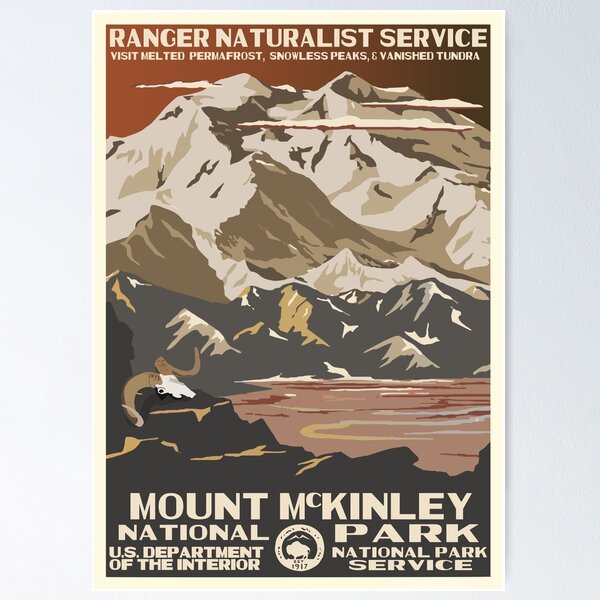This vintage-style poster, reminiscent of the 1940s or 1950s, features a color image that captures the dramatic landscape of Mount McKinley National Park. The background showcases a sky adorned in varying shades of brown, darker on the right and lighter on the left, suggesting a transition from night to dawn. Dominating the scene are stately mountains depicted in a palette of white, brown, beige, and gray, with the sun illuminating the left sides in yellowish tones. White clouds hover above the peaks, adding a touch of ethereal beauty to the composition.

Central to the design is a rugged, rocky foreground, leading the eye to a body of water that strikingly blends hues of red, pink, and yellow. Text at the top of the poster reads "Ranger Naturalist Service" in bold white letters, along with the subtext, "Visit melted permafrost, snowless peaks, and vanished tundra," inviting viewers to explore the altered natural wonders of the park. At the bottom, more text in white announces "Mount McKinley National Park," flanked by "U.S. Department of the Interior National Park Service." A noteworthy detail is a logo situated in the lower center, featuring a buffalo and the year "1917," further enhancing the poster's historical charm.